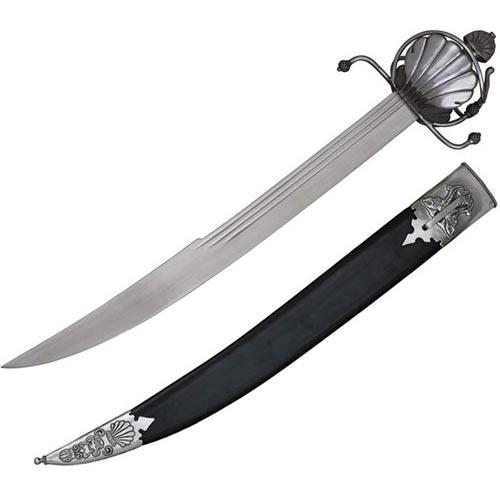The image showcases a meticulously crafted sword displayed above its matching scabbard, all against a plain white background. The sword, forged from silver metal, features a hilt and handguard that gleam with the same metallic sheen. The hilt is partially visible, revealing a half-circle design intricately engraved with what appears to be a rising sun motif. The handguard is elaborately shaped like an open seashell, encapsulated by a metal ring, with extensions flaring out to the sides to complete the guard. The blade itself has three subtle grooves running halfway along its length, adding to its elegance and craftsmanship. Below the sword lies the scabbard, made of narrow black leather accented with silver metal tips. The bottom of the scabbard mirrors the seashell design found on the handguard, creating a cohesive appearance. Additionally, the upper metal tip of the scabbard is adorned with a functional belt loop, completing the set’s beautifully unified aesthetic.